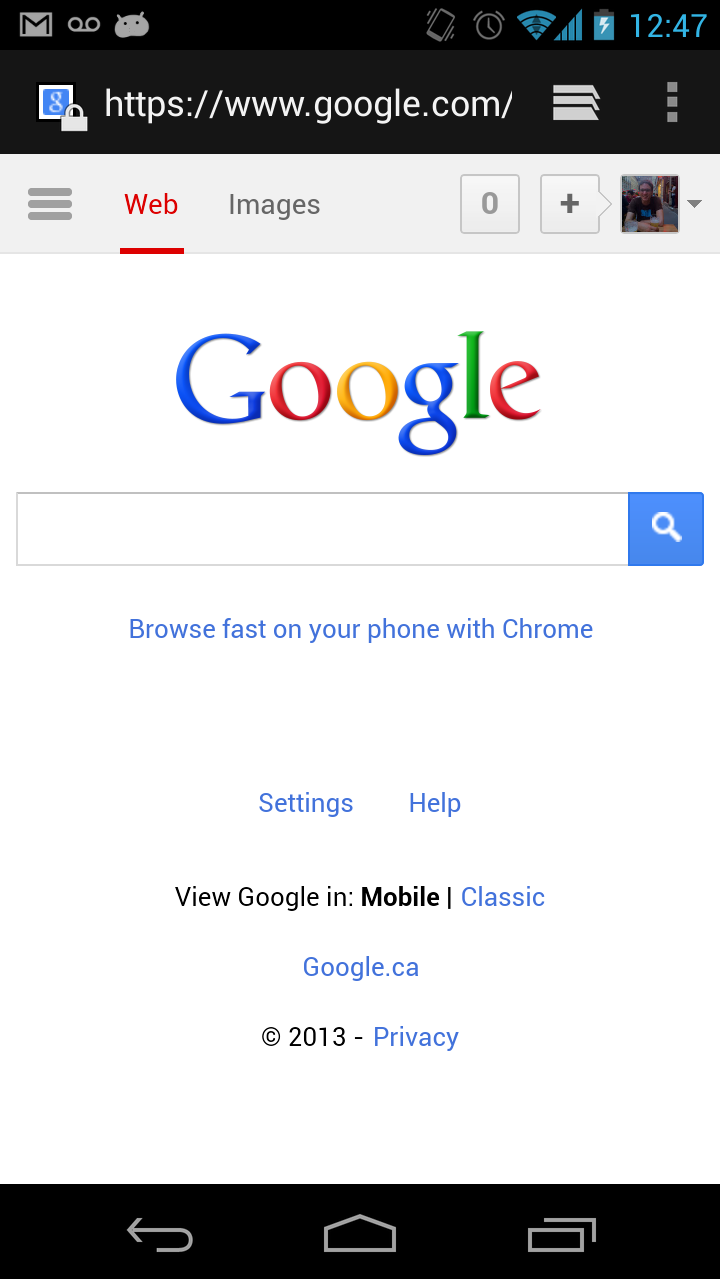The screenshot captures an older Android phone displaying the Google homepage. In the top left corner of the screen, there are several small notification icons, including Gmail, voicemail, and a system Android icon. The time is displayed as 12:47. The Google homepage is displayed prominently on the screen, with the recognizable Google logo at the top. Below the logo is an empty search bar. Directly beneath the search bar is a blue caption that reads, "Browse fast on your phone with Chrome," followed by options for "Settings" and "Help." Further down, there are links to view the site in either mobile or classic mode. At the very bottom, the text reads "Google.ca 2013" and "Copyright 2013." The bottom row of the screen features the standard Android navigation buttons: a back key on the left, a home key in the center, and an app drawer key on the right.